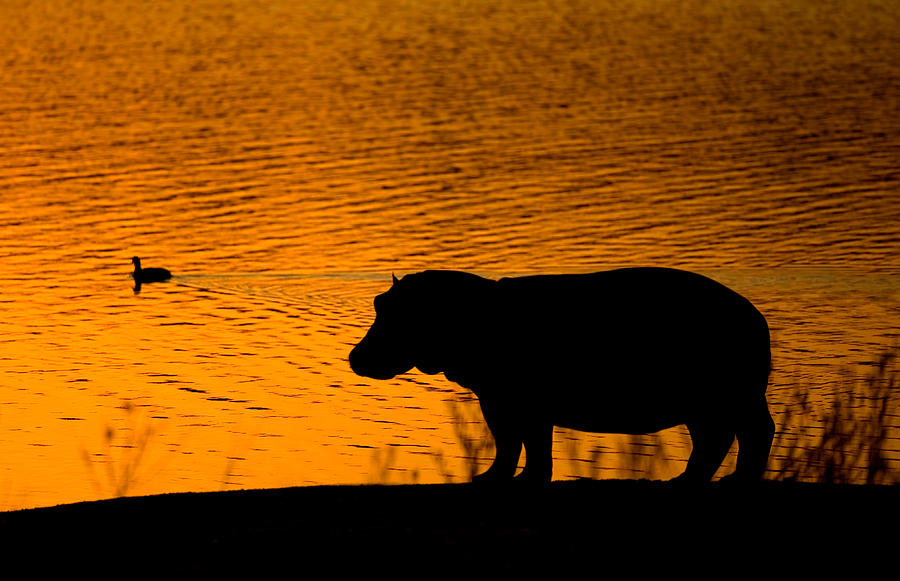In this professionally captured sunset photograph taken outdoors, the silhouette of a majestic hippopotamus stands prominently at the edge of a rippling, golden-hued body of water. The hippopotamus, outlined starkly in black, is framed by tall, dark silhouettes of reeds and grass. To the left, the black shape of a duck floats peacefully on the shimmering, orange-tinted lake, providing a serene contrast to the dark silhouettes in the foreground. The scene is lit by the dark red ember-like glow of the setting sun, casting a striking reflective light across the water surface. The slightly hilly ground beneath the hippo further accentuates the natural setting of this tranquil moment.